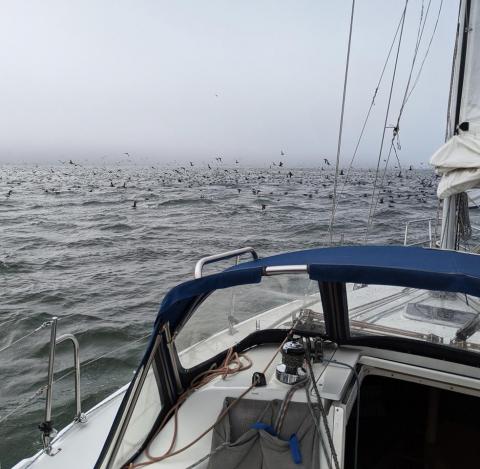This photograph captures a serene outdoor scene from the aft of a white sailboat with blue trim, floating on a choppy, gray body of water. The overcast, foggy sky above fades from a pale blue at the top to predominantly white. The background hints at a faint, gray mountain range, barely visible through the mist. The horizon is bustling with hundreds of birds, some soaring low in the sky, while others skim the water's surface, possibly hunting for fish below. The right bottom of the image reveals part of the sailboat's interior, featuring some wirings or strings and a rail. A gray bag hangs from the boat's side, and a blue tarp covers part of the deck. The image conveys a sense of calm and stillness, with no crew members in sight on the approximately 25 to 30-foot sailboat.